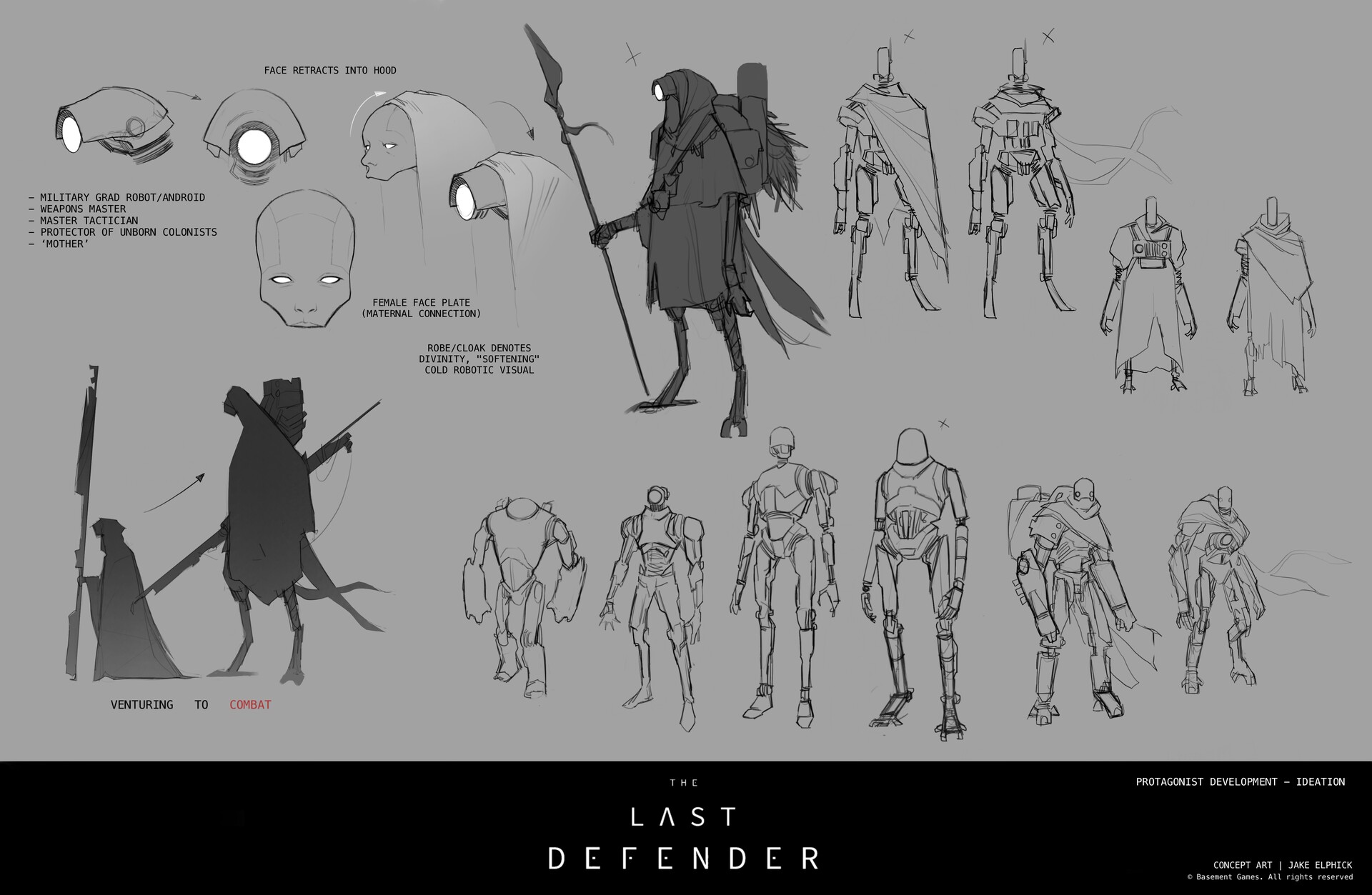This is an illustrated guide for the character "The Last Defender," potentially designed for an animated movie, computer game, or science fiction narrative. The majority of the image is set against a gray background, and it is meticulously organized to show various conceptualizations of the character. In the top left corner, there are detailed close-up designs of the character's head and face, demonstrating how the face retracts into a hood. In the center at the top, a dark gray drawing depicts the character standing and staring off to the left, clad in a cloak and carrying a staff with a flag attached. To the right of this, in the top right corner, line drawings meticulously outline the character's details with and without the cloak, providing views of different angles and clothing configurations. The bottom left corner features silhouette shots capturing the character's movement and weapon stance, while the bottom of the image presents various designs for the character's armor and mechanical elements. Across the very bottom, a prominent black stripe bears the title "The Last Defender" in white text, along with the smaller, hard-to-read text "Protagonist Development Ideation," indicating this is a conceptual design board guiding the character's development in different settings, angles, and with different accessories.